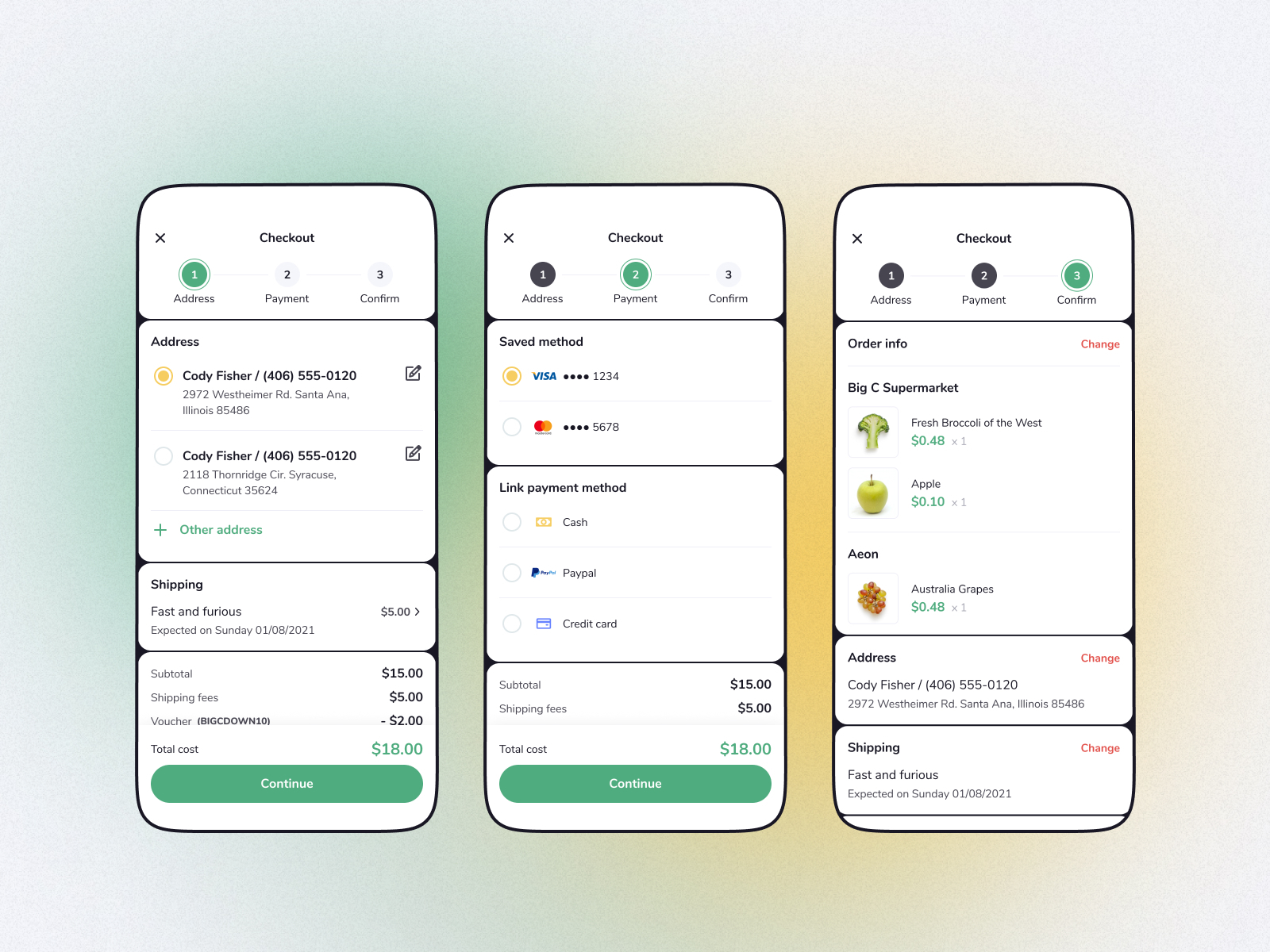Caption: "In this image, we see a detailed confirmation of a recent online purchase. The order includes 3 smartphones and 2 light shows, all set to be shipped to Cody Fisher at 2972 West Timer Road, Santa Ana, Illinois, 85486. The payment has been confirmed, and six different checkout addresses were involved in the transaction. For any inquiries, Cody Fisher can be contacted at 406-555-0120."